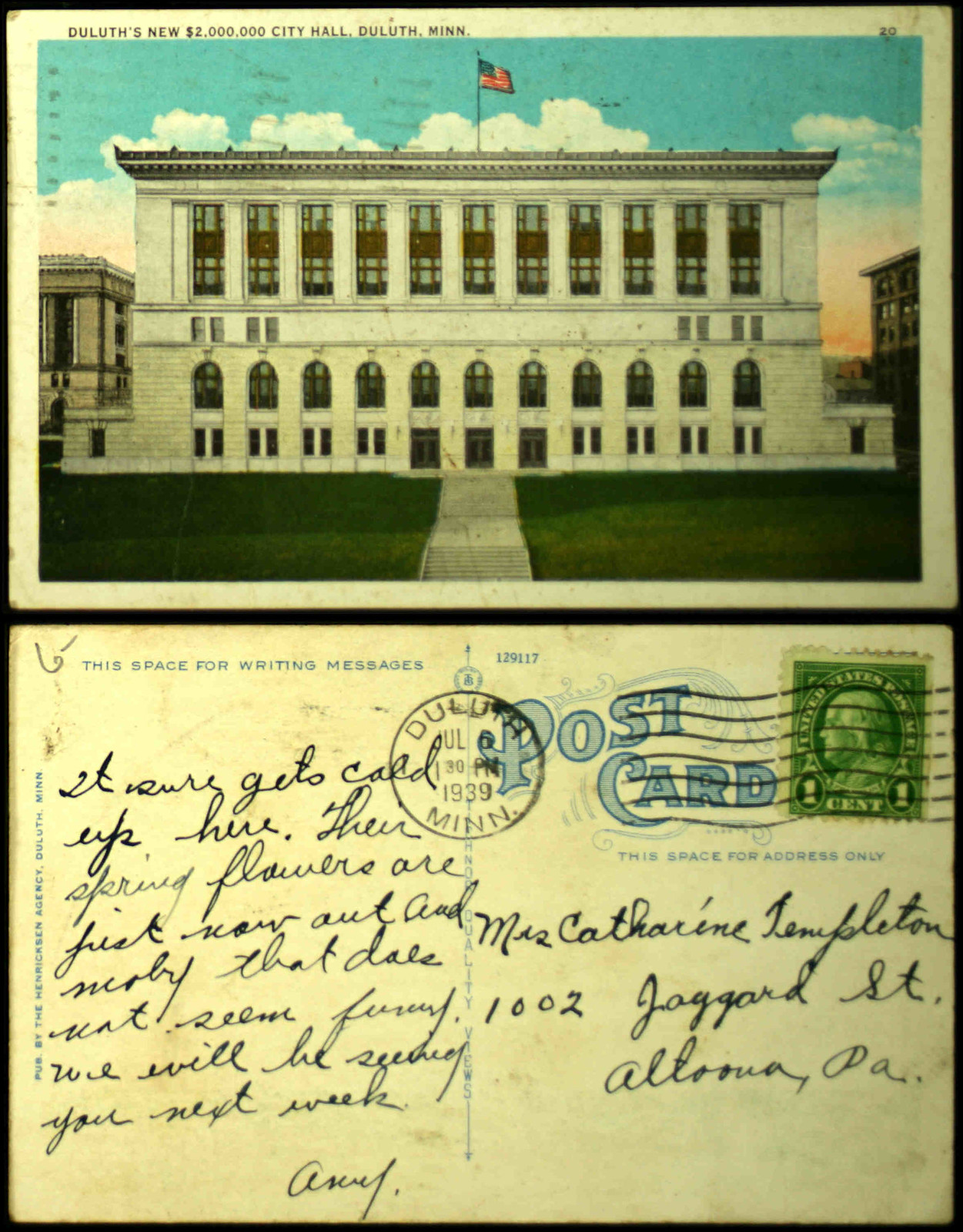This image appears to be a vintage postcard showing both the front and back. The front features a painting of a monumental administrative building identified as Duluth's new $2 million City Hall in Duluth, Minnesota. The building, which is two or three stories tall, is depicted with large vaulted and rectangular windows, with the arched ones being more decorative on the ground floor. The architecture features a flat roof crowned with an American flag centered at the top, fluttering rightward against a blue, slightly cloudy sky. A white stairway leads up to the building through a grassy foreground.

The postcard retains its antique charm with visible yellowing, minor scratches, and brownish discoloration, suggesting its considerable age. The caption at the top of the front side reads: "Duluth's new $2 million City Hall, Duluth, Minnesota".

The back of the postcard carries a one-cent stamp, which possibly features Benjamin Franklin, and is postmarked "Duluth, July 6, 1939, Minnesota." The sender, addressing Mrs. Kathleen Templeton in Pennsylvania, writes in cursive, mentioning the cold weather, late-blooming of spring flowers, and a promise to see the recipient next week. The handwritten message, though difficult to decipher due to its heavy cursive script, spans most of the left and right sections. The back also includes printed text: "This Space for Writing Messages" on the top left and "Postcard" on the top right, punctuated by horizontal squiggly lines as part of the postmark. The postcard's aged condition is further accentuated by visible stains, especially on the left side.